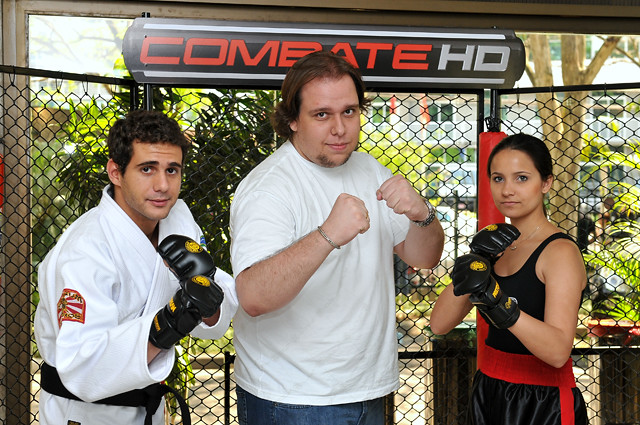This photograph captures three individuals, assumed to be mixed martial arts (MMA) fighters, standing outdoors on a sunny day in front of a black cage-like fence with houses and greenery visible in the background. Above the cage hangs a black banner with white borders and bold red text that reads "Combat" followed by a chromish white "HD."

The person on the far left is a man wearing a traditional martial arts gi—a white robe suit—with a red patch on the right arm, a black belt, and black and yellow sparring gloves. He stands in a fighting pose, fists up and ready to spar.

In the center is a significantly taller and larger man who contrasts with the other two. He is dressed in casual attire: blue jeans, a white t-shirt, bracelets, and a watch. Despite his casual clothing, he also holds up his fists in a sparring stance.

On the far right is a smaller-framed woman with darker skin. She wears a black tank top, black and red silk shorts, and black and yellow fighting gloves, similar to the man in the gi. Like the others, she stands in a fighting pose, ready for combat. This detailed snapshot exudes the spirit of mixed martial arts, depicting readiness and diverse participants.